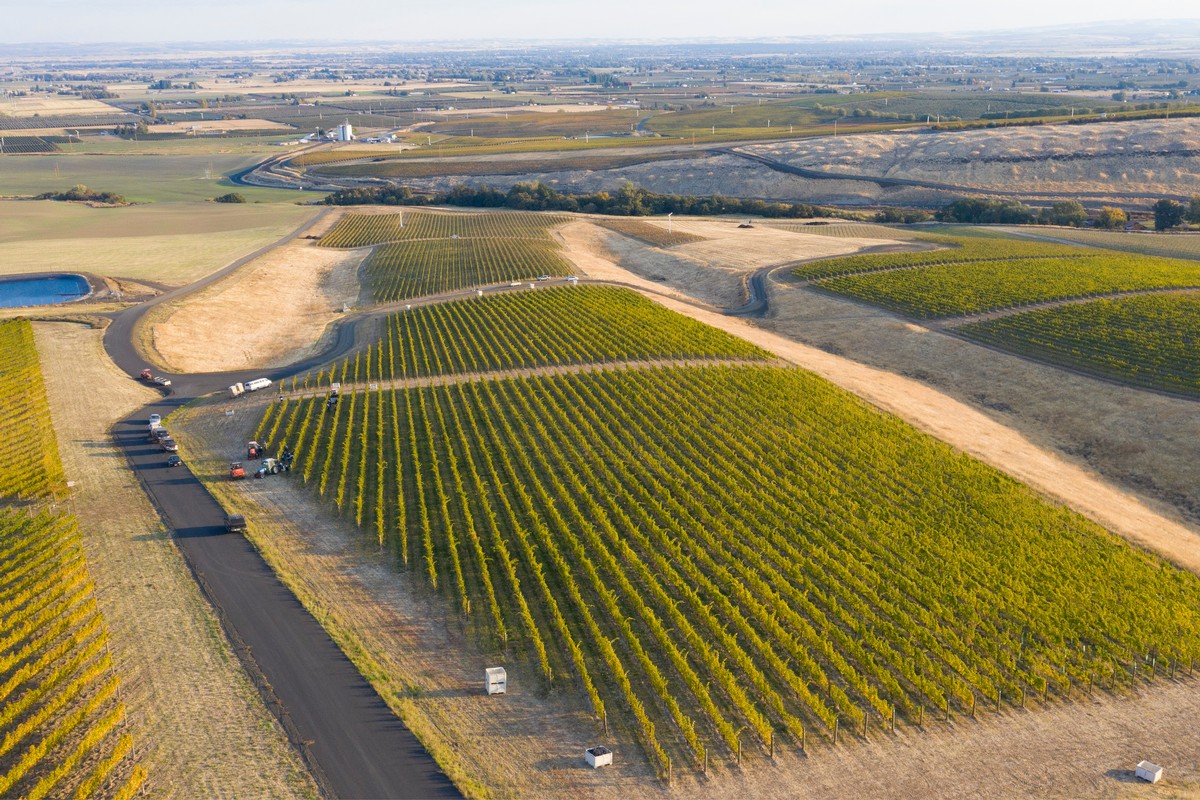This aerial photograph captures a sprawling vineyard, meticulously arranged with approximately 40 to 50 rows of lush green vineyard plants, all organized in neat, orderly sections. The layout includes four primary field sections divided by paved roads, where several harvesting vehicles and machinery are visible. Scattered white container boxes likely serve as storage for the harvested grapes. Adjacent to the vineyards, irrigated farmland and other agricultural fields extend into the distance, intersected by additional sandy pathways. To the left, a visible blue pool of water stands out against the earthy landscape, although it appears artificial. The background reveals hints of a town or grain silo towers and more expansive farm fields, partially obscured yet adding depth to the scene. Overall, the photograph melds the structured beauty of viticulture with the broader agricultural setting under a sunny, clear sky.